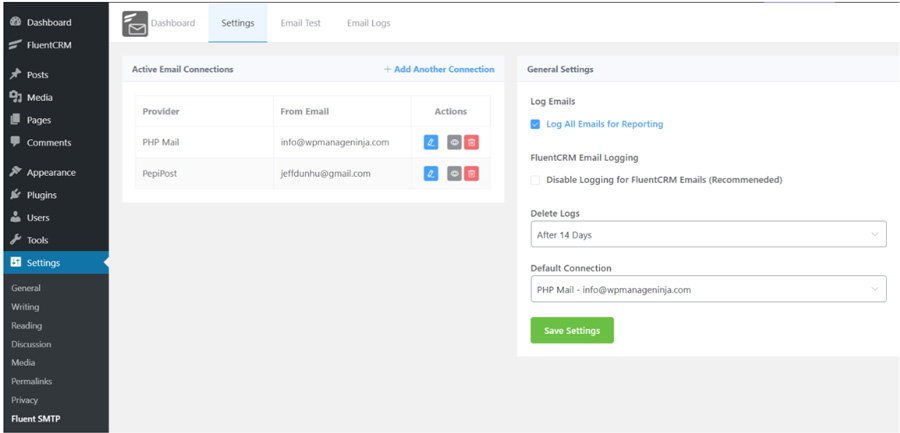The image captures the interface of an application dashboard featuring a pale-colored background. On the left side of the screen, there is a black vertical sidebar with white text displaying various options: Dashboard, Fluency RM, Posts, Media, Pages, Comments, Appearance, Plugins, Users, Tools, and Settings. The 'Settings' option is highlighted with a blue horizontal bar. Beneath the 'Settings' tab, a submenu displays additional options including Generals, Writing, Reading, Discussion, Media, Panel Links, Privacy, and Fluent SMTP. 

To the right side of the screen, there are two prominently visible windows. The first window on the left is labeled 'Active Email Connections,' while the adjacent window on the right is labeled 'General Settings,' providing further configuration options for the application. The clean layout ensures easy navigation and quick access to various functionality within the application.